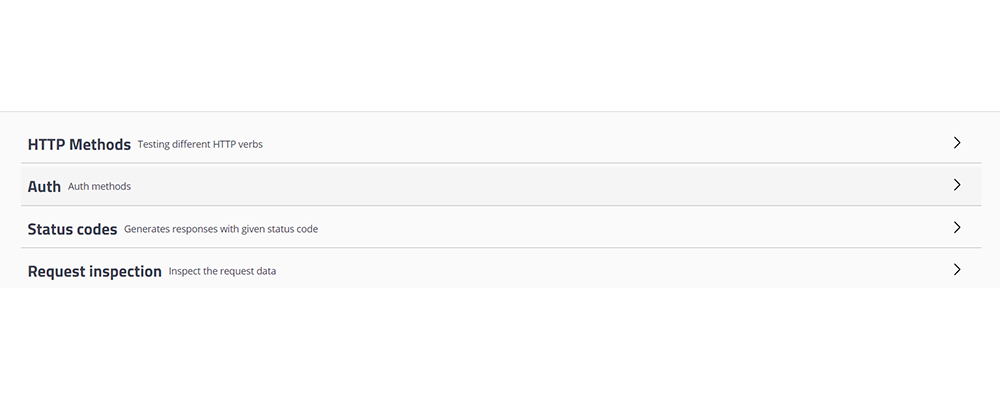Here is a detailed and cleaned-up caption for the image:

---

This digital image from my website features a well-structured list of HTTP testing tools and options. At the top left, in bold black font, is the heading "HTTP METHODS," with an explanatory subtext in regular font: "Testing different HTTP verbs." Adjacent to these, on the right side of the image, is a clickable button. 

Directly below, the text "AUTH METHODS" appears in bold black font, accompanied by a grey subtext: "Off methods." Beneath this, another heading "STATUS CODES" is displayed in bold black font, with a subtext in grey font: "Generates responses with given status code," followed by a right arrow icon to its right.

The final line showcases the heading "REQUEST INSPECTION" in bold black font, along with the explanatory subtext in regular grey font: "Inspect the request data."

---

This refined caption offers a comprehensive description of the image while maintaining clarity and detail.